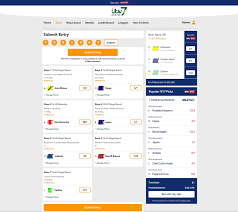The image appears to be a low-resolution screenshot of a website, making the text unreadable due to blurring when zoomed in. The website has a predominantly gray background with a blue border at the top, which also features a small section of white space and a logo that includes the number '7,' although the exact text is indiscernible. Below the blue border, there is a navigation menu with seven buttons, one of which is highlighted in orange, suggesting it has been selected, while the others remain black. An icon resembling a person, likely representing user profile access, is positioned slightly to the right of the center in the second line. The main content area follows, divided into multiple sections: three columns of white boxes in the first row, followed by four and then three boxes, and finally, two columns in the last row. These boxes appear to contain various elements, though the details are unclear. The design features sporadic use of orange, particularly for buttons and accents, with one of the boxes being bordered in blue at the bottom and on the sides. Despite the blurred text, the visual structure and color scheme hint at an organized and interactive web page layout.